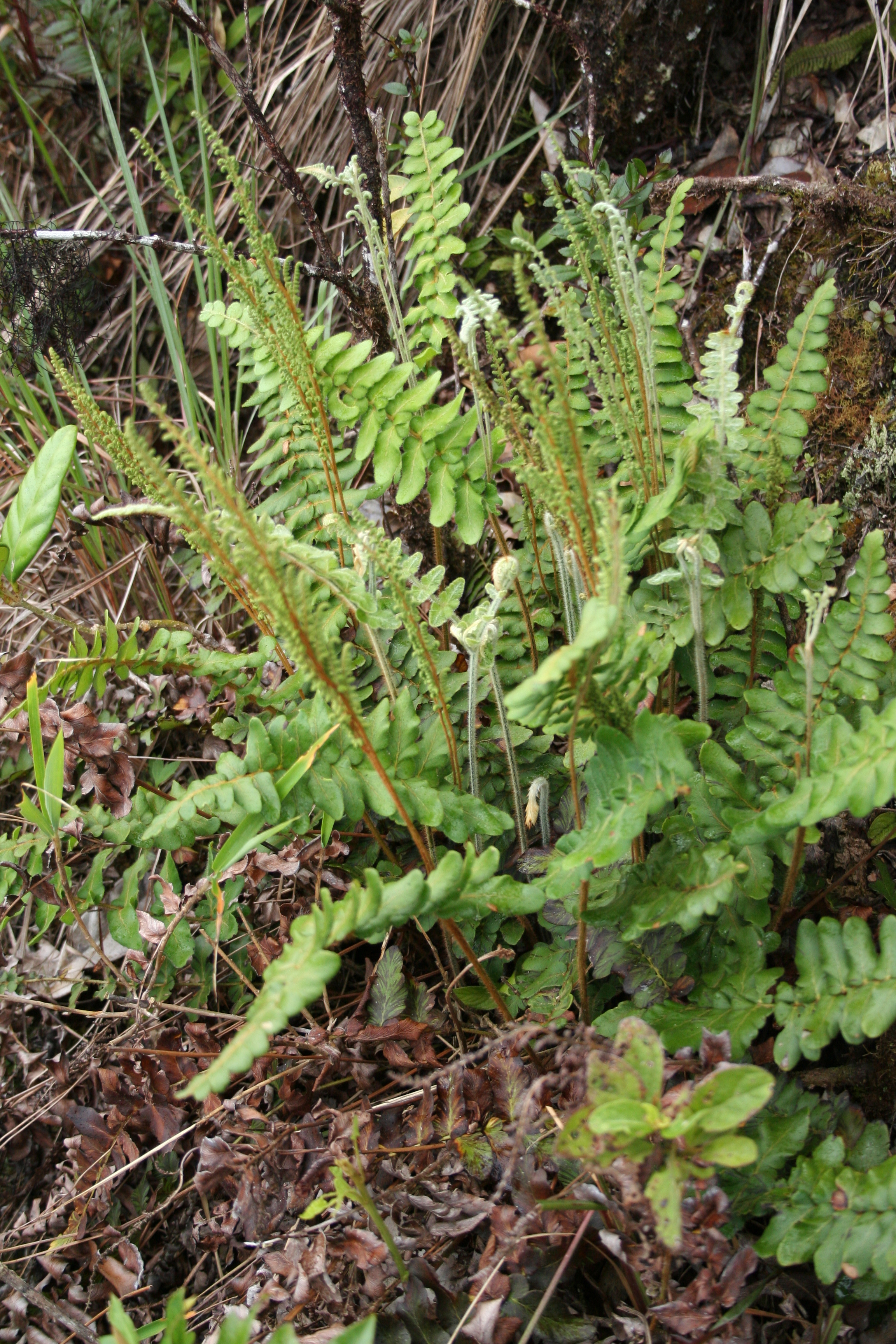The image presents a close-up scene of a tall, weedy plant amidst a dense, natural setting. The focal point is a brown-stemmed plant with circular green leaves, standing tall amidst a backdrop of brown, straw-like hay and dead leaves. Surrounding the main plant, the ground is littered with various shades of brown and green foliage, twigs, and sticks, alongside some black spots that resemble holes in the ground. Interspersed among the plant's leaves are other tall, hay-colored stalks with fuzzy tips. The photograph appears slightly out of focus, with finer details blurred, especially in the foreground, while the background remains somewhat clearer. This outdoor nature scene captures a mix of vibrant and decaying elements, illustrating a raw, unkempt ambiance typical of a wild, grassy area.